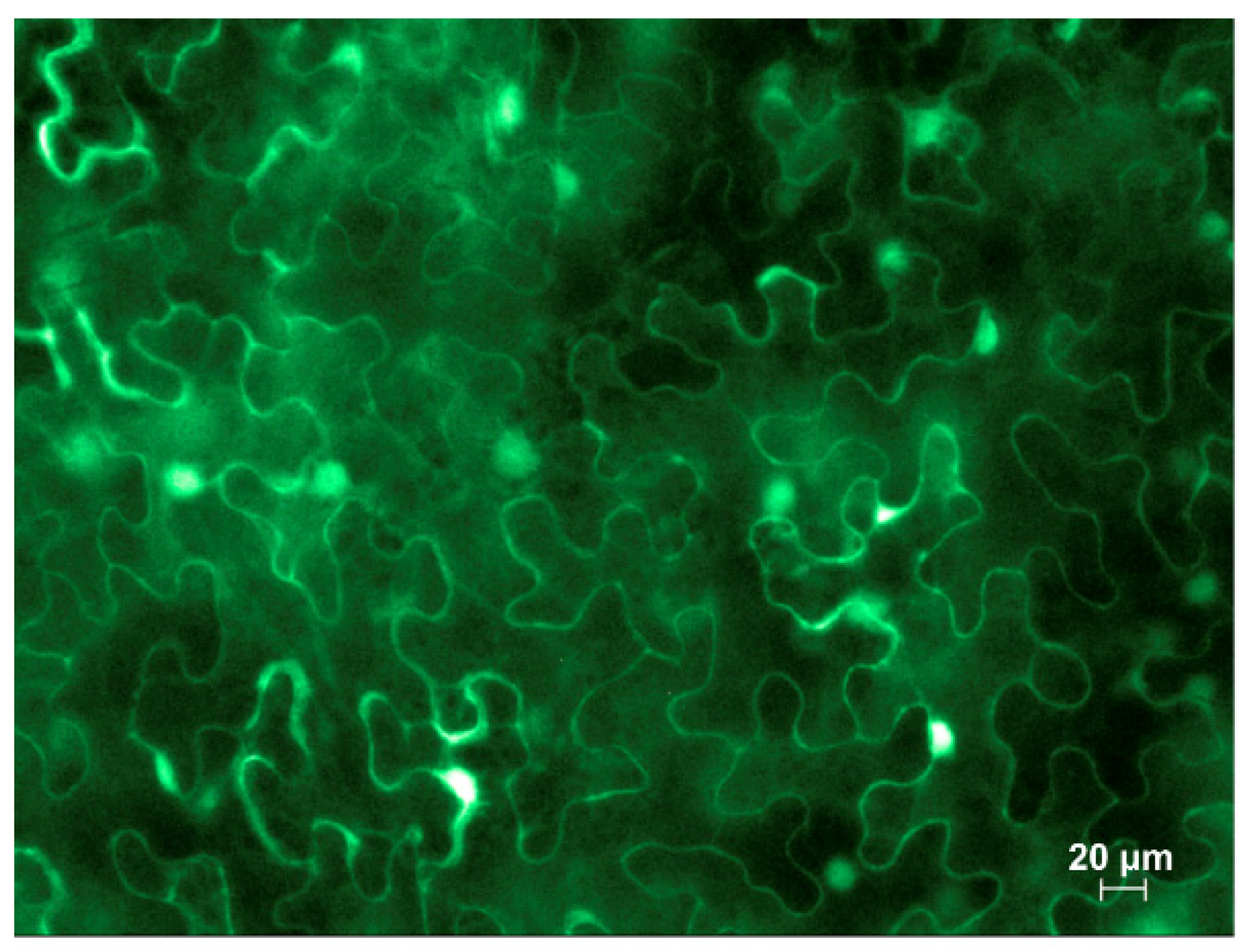The image depicts a microscopic view featuring various shades of green, ranging from bright neon to dark, all set against a predominantly dark, blackish background. The scene is filled with wavy, swirly lines and abstract shapes that appear to glow with an almost luminescent quality, creating a vibrant contrast against the darkness. Some of these green lines and shapes are more pronounced, while others are faint, blending into the hazy, fog-like areas of green. The edges of these shapes are slightly blurry, adding to the sense of depth and texture. In the bottom right corner of the image, the text "20 UM" is visible, indicating a scale of measurement often associated with microscopic imaging, possibly from an electron microscope.